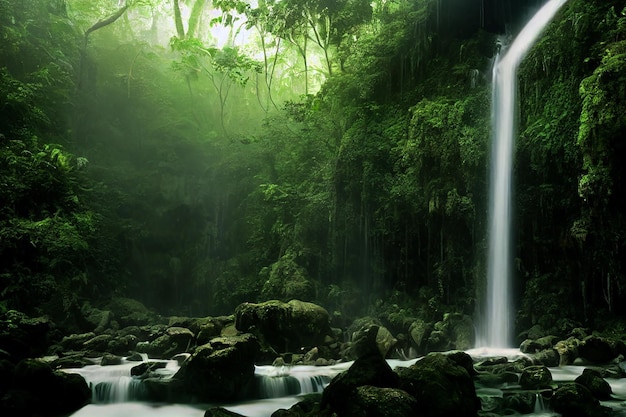The image captures a densely lush jungle scene, dominated by rich green foliage cascading over a cliff edge. A narrow, straight waterfall flows from the top right-hand corner, descending dramatically into a rocky area below. The rocks, covered in moss, form a flat surface where the water trickles and pools. The scene is textured with varying shades of green, from the dark greens of the dense foliage hanging near the waterfall to the lighter greens and whites in the upper left-hand corner, suggesting a glimpse of the sky. Despite the spot of light from above, the dense canopy allows only minimal light to penetrate, giving the overall scene a deep, verdant appearance. The waterfall appears blurred in the photograph, capturing its motion as it streams down, creating a stark white contrast against the green and brown hues of the surroundings.